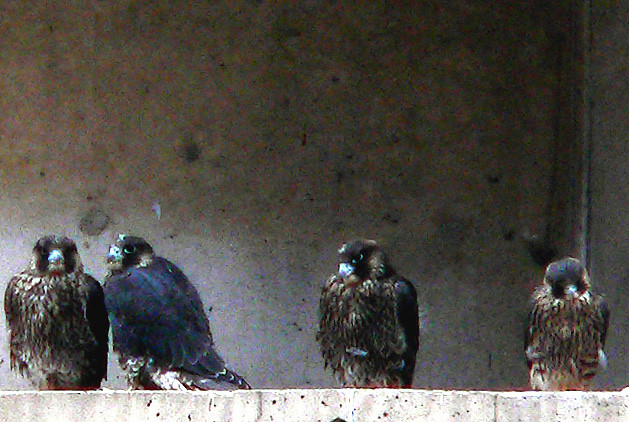In this grainy photograph, four juvenile hawks perch on the ledge of a man-made structure, possibly cement, set against a mottled tan and black background. The hawks' dark heads and backs contrast starkly with their heavily streaked and barred light bellies. Their plumage appears rough and ragged, as though they are molting. The birds and the background exude an almost surreal, Photoshopped quality. On the far left, one hawk faces the viewer directly. Next to it, another hawk's body is turned inward while its head and sharp, dark eyes rimmed with white look towards the camera. The third hawk also faces forward, displaying its streaked breast, and the fourth, positioned furthest on the right, similarly looks towards the camera with a dark intensity. The hawks' yellowish and black feathered undersides contrast with their brown-tipped beaks, sitting in a seemingly artificial but intriguing setting.